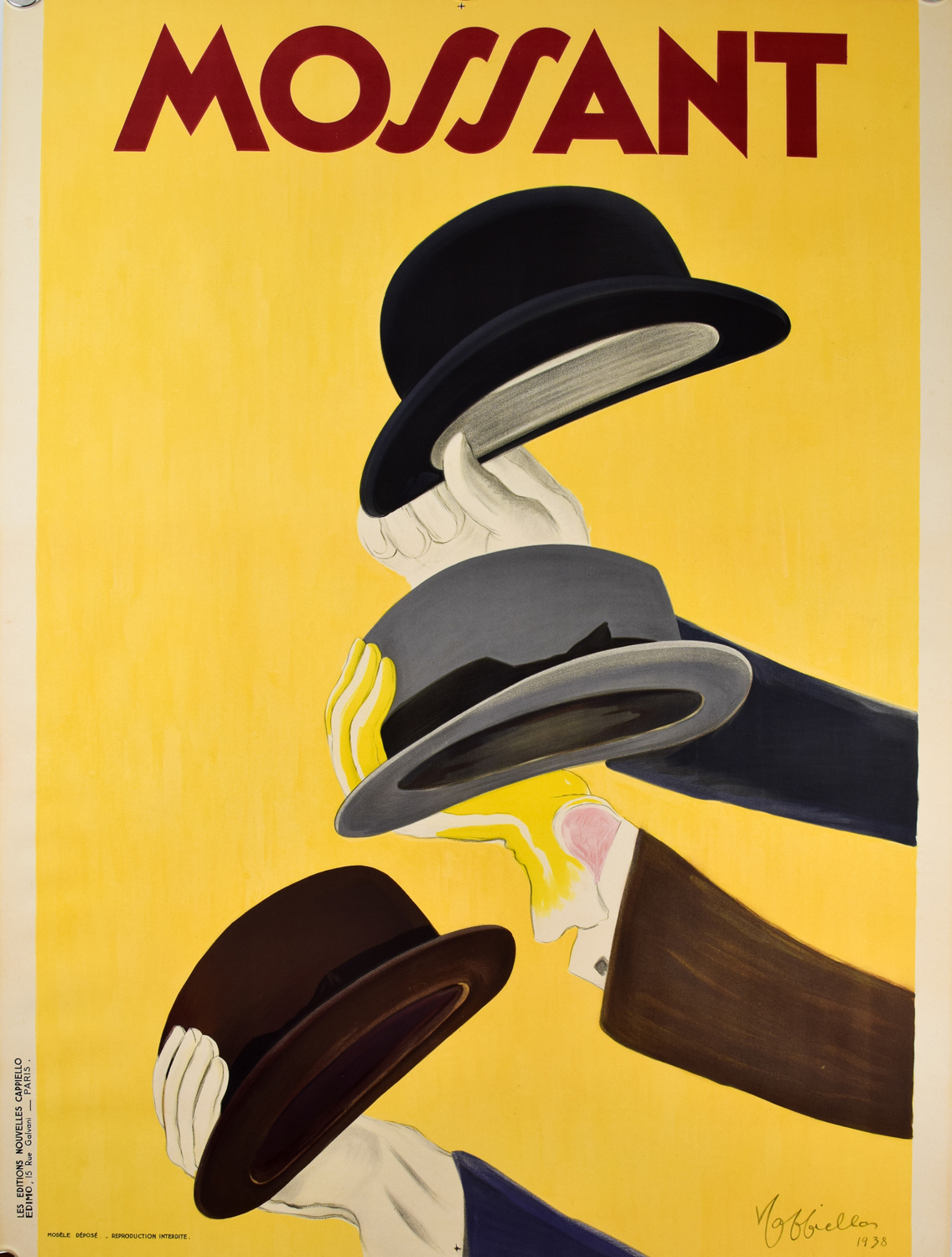This is a detailed painting-turned-poster with a primarily yellow background bordered by beige on either side. Centering the composition are three hands extending from the right, each holding a differently styled hat, stacked vertically. The topmost hat is a black bowler being held by a hand in a white glove with a blue sleeve. Below it, the middle hat is gray with a black band, held by a hand in a yellow glove with a brown sleeve. The bottom hat, brown in color, is held by a hand in an off-white glove and a blue sleeve. 

At the top of the poster, the text "Mossant" is prominently displayed in dark maroon, more abstract font. The artist's signature is visible at the bottom right, dated 1938. On the left side, additional text reads: "Les Editions Nouvelles, Cappiello," indicating its likely French origin.